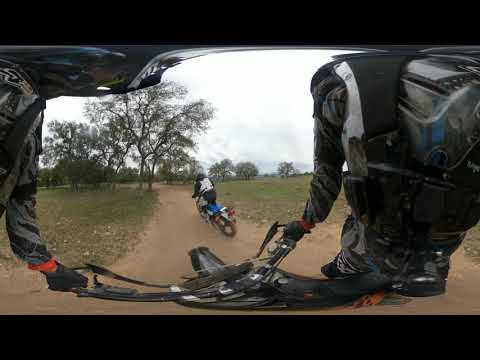In this image, we observe an outdoor scene likely set in the middle of the day on a dirt bike track. Dominating the foreground is a motorcyclist riding down a dirt path, which is surrounded by patches of grass on both sides. The rider is dressed in a black uniform with a white vest and helmet, riding a bike with a dark blue seat and a silver rear section. 

Two men, also in protective gear and possibly uniforms, occupy the lower part of the image, lifting a fallen motorcycle—one using his right hand, the other his left. Trees of varying heights line the horizon, leading up to the cloudy, bluish-white sky. The palette includes colors such as black, gray, white, green, orange, red, tan, and silver, lending a detailed richness to the scene. 

Framing the view, there are elements that give the impression of looking through a vehicle window, adorned with futuristic or robotic cables and twisted cloth-like materials hanging down, possibly monitoring the race. 

Overall, the image captures a dynamic and multi-layered outdoor moment centered on the activities and surroundings of a dirt bike course.